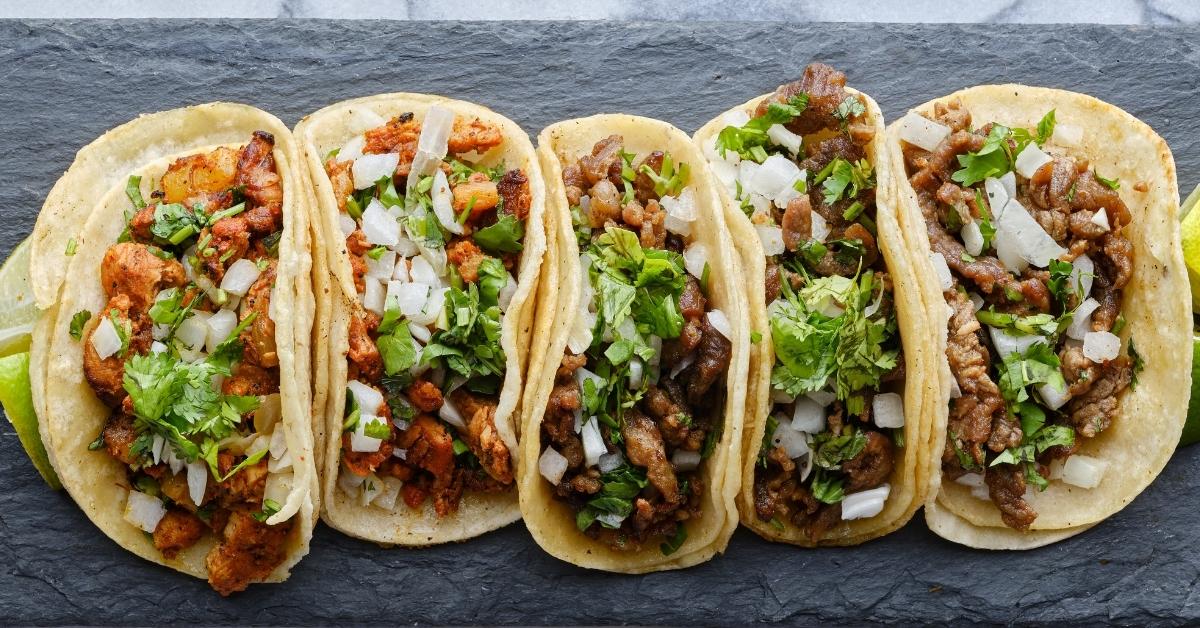This color photograph, taken in landscape orientation and viewed from above, showcases a mouth-watering lineup of five artisanal soft tacos displayed side by side on a gray slate surface. Each taco is nestled in double shell wrappers, with lightly toasted tortilla shells that exude a freshly made appeal. 

Arranged in a visually appealing row, the leftmost taco is garnished with a lime wedge tucked underneath, adding a vibrant touch to the presentation. The fillings appear to be a mix of chicken for the first two tacos, while the remaining three seem to be stuffed with steak or carnitas. The tacos are generously topped with a blend of chopped white onions and green cilantro leaves, lending a burst of color and freshness to the dish. 

The photograph's detailed realism emphasizes the artisanal quality of these tacos, highlighting the appetizing blend of brown, green, and white hues, and capturing the essence of gourmet street food.